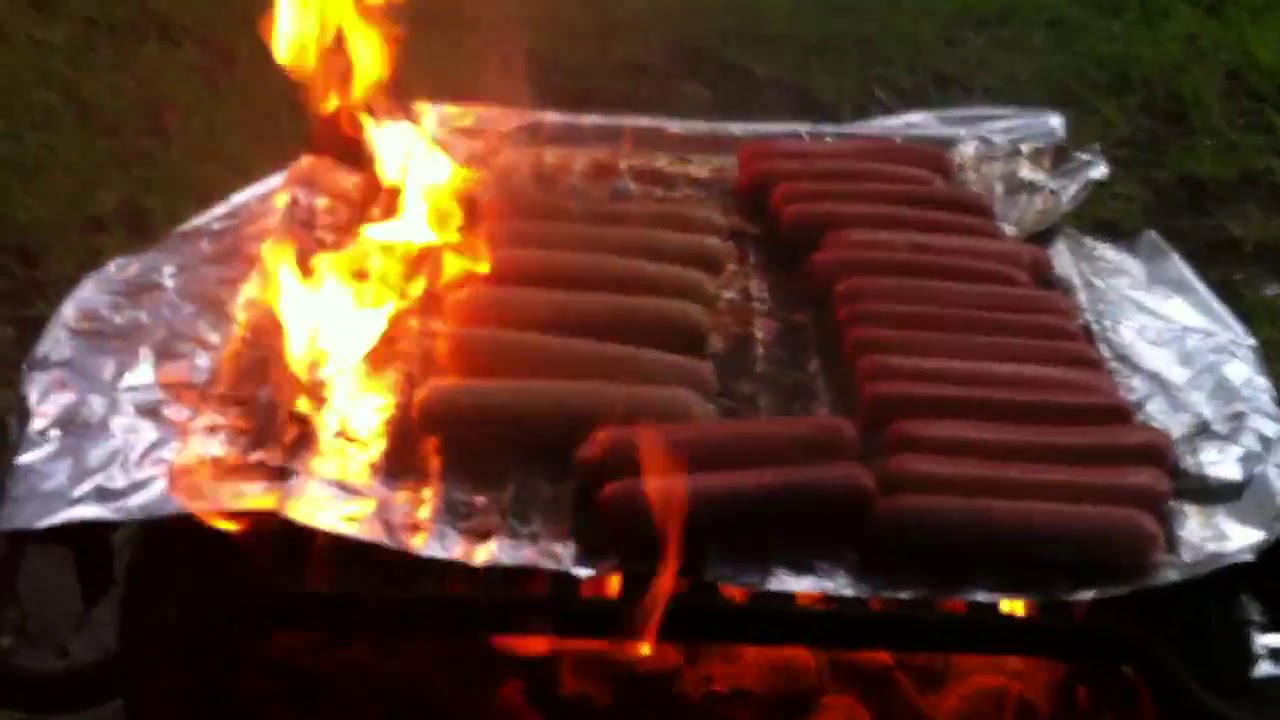In this image, we see an outdoor scene featuring a black grill positioned on a grassy field, likely in a park setting. The grill is covered with a sheet of aluminum foil, through which flames are visibly rising on the left side, fueled by glowing red embers underneath. Arranged neatly on the foil are approximately 22 cylindrical meat items, predominantly hot dogs with some possibly being sausages. These items, reddened by the heat, are in the process of being cooked. The scene is set either in the early morning or late evening, as the light is dim, adding a cozy atmosphere to this outdoor grilling session.